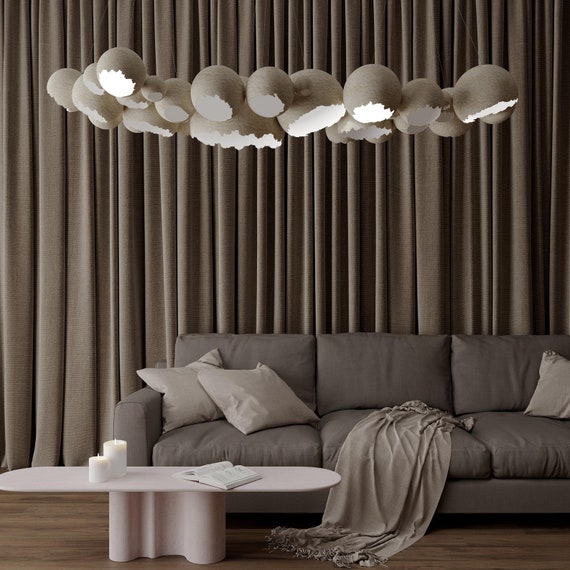The image portrays a sophisticated, modern living room set in a monochromatic style. The centerpiece is a plush, gray sofa with three seat cushions and three back cushions, complemented by light gray throw pillows and a fringed light gray shawl draped casually over the middle cushion. Positioned in front of the sofa is an elegant, minimalist coffee table with a sleek, white, surfboard-shaped top resting on a central pedestal. On the table are two white pillar candles and an open book, adding subtle decorative touches.

Suspended above the sofa is a unique, modernistic chandelier composed of horizontal arrays of half-circle elements. These elements resemble broken eggshells with jagged edges and emit a warm light from within, enhancing the room's ambiance. The backdrop features a floor-to-ceiling curtain in a densely pleated, grayish-brown fabric that seamlessly blends with the monochromatic tones of the room.

The living room is set on a grayish-brown hardwood floor, further contributing to the cohesive color scheme of various shades of gray, brown, and white. This well-composed photograph captures the stylish elegance and modern design of the living room, likely intended for a furniture or interior design marketing campaign.